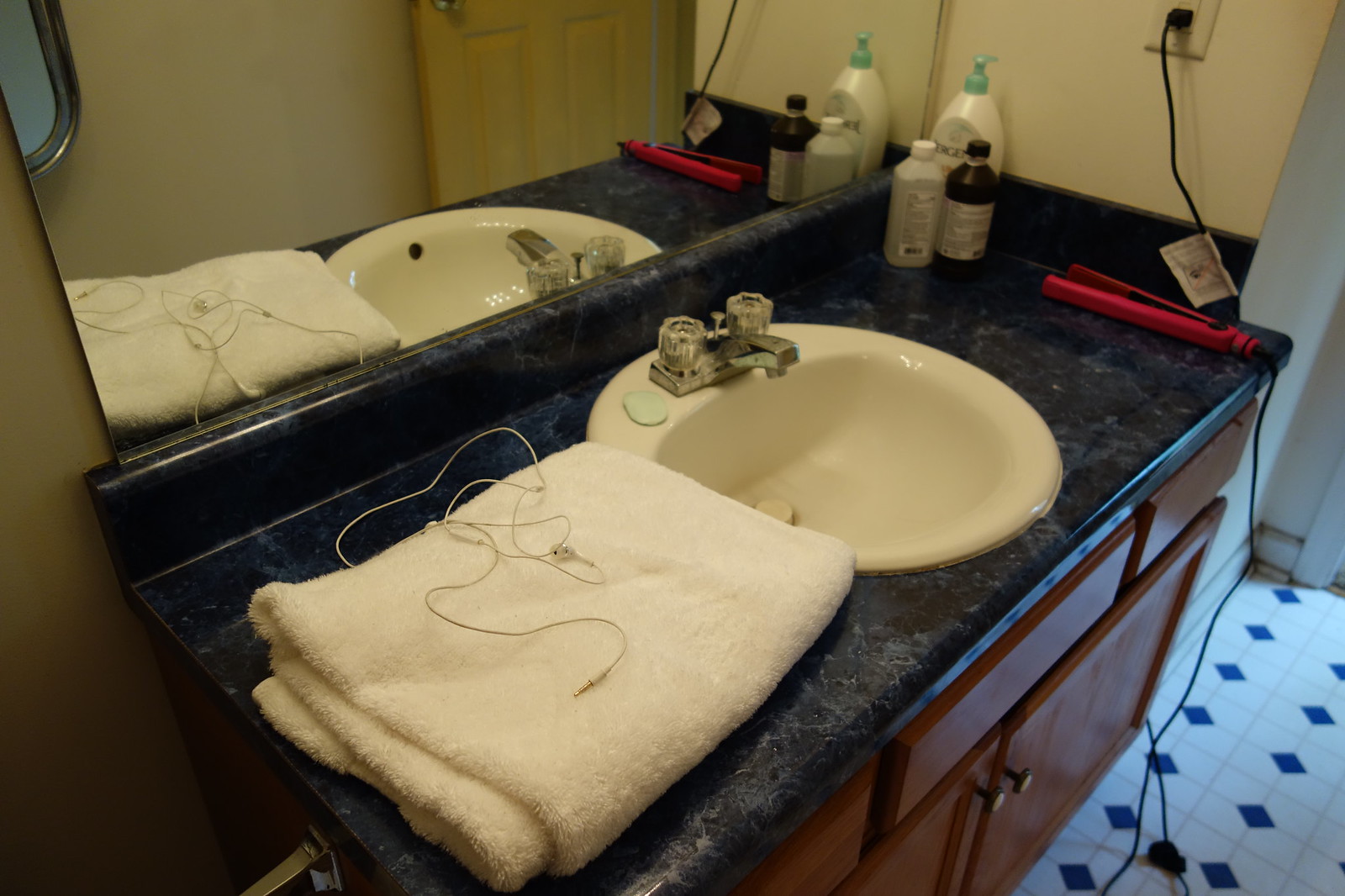The photograph depicts a modest bathroom with a functional yet unadorned aesthetic. The centerpiece is a black faux marble countertop, complete with a built-in splash guard that extends along the back and partially along the sides. The walls are a light tan or whitish color, seamlessly crafted from drywall, suggesting a standard residential build rather than a mobile home.

The short wall directly behind the sink features a single electrical outlet, occupied by a black plug with a cord that traces down to the floor and back up, connecting to a red hair straightener resting on the counter. To the right of the sink are three bottles, containing lotion, alcohol, and peroxide, respectively. A neatly folded white towel sits to the left of the sink, beside which lies an enigmatic white device with an electric cord and what appears to be a coaxial cable, possibly an earphone.

A small blue bar of soap is positioned to the left of the stainless steel faucet, which sports clear plastic handles. The faucet and handles, although designed to mimic stainless steel, are actually plastic with a nickel-plated finish. The white sink basin is simple and functional, mirroring the utilitarian theme of the space. 

Above the sink hangs a plain contractor's mirror, devoid of any decorative features. The floor is covered in a familiar black and white checkered vinyl, a classic design choice that adds a hint of nostalgia to the otherwise straightforward bathroom.